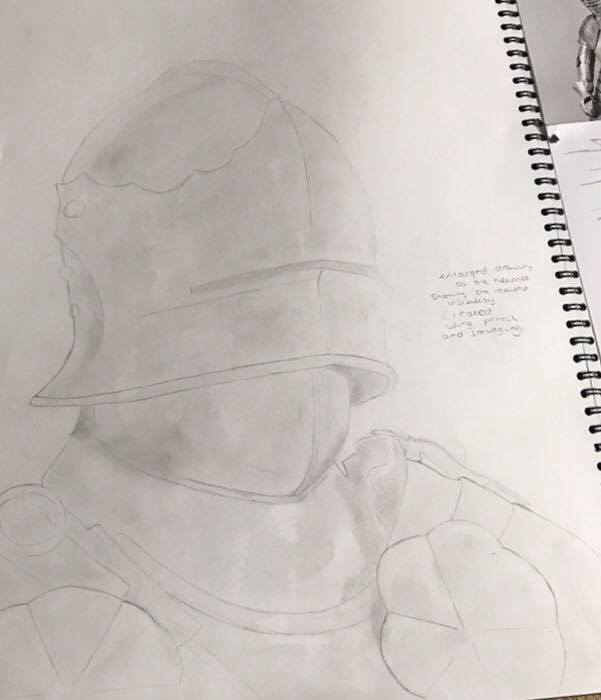A highly detailed sketch of a medieval soldier's manual is depicted, characterized by meticulous illustrations. The central figure wears a robust metal helmet adorned with distinct rivets. The body armor appears to be crafted from metal, extending seamlessly from left to right, enhancing the soldier's fortified appearance. On both sides of the armor, stylized petals or ornamental designs are visible, adding a touch of artistic flair. To the right of the sketchbook page, there are bindings, suggesting the document's functional purpose. Scattered letters and partially readable text are inscribed across the sheet, contributing to the historical and educational essence. The intricate bread-like section is identified as another segment of the metal armor, underscoring the attention to detail in this captivating manual.